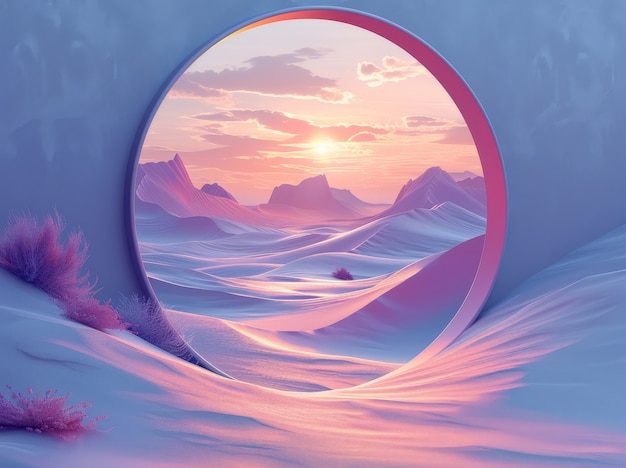A captivating image features a circular cutout in a wall, revealing a beautifully serene sunset sky. The sky is illuminated with soft, warm hues of pink and peach, giving it a dreamy, ethereal quality. Wisps of delicate clouds scatter across the scene, enhancing the tranquil ambiance. The circular frame in the wall perfectly captures this peaceful moment, making the vibrant, glowing colors of the sunset stand out vividly against the silhouette of the cutout.